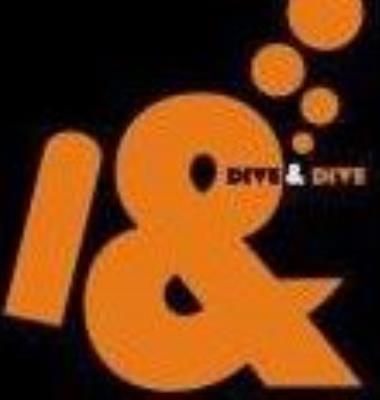The image is a pixelated depiction of a logo or album cover with a predominantly black background. Dominating the foreground is a large ampersand symbol in light orange color. Adjacent to the ampersand is a vertical orange line, rounded at one end and straight at the other. In the top right corner of the image, there are four progressively larger orange bubbles, each increasing in size as they ascend. Superimposed on the large orange ampersand is the word "Dive," rendered in black text. Below this, there is a smaller white ampersand symbol, followed by the word "Dive" in orange text. The combination of these elements suggests the logo reads "Dive & Dive," although the pixelation makes the text slightly difficult to discern.